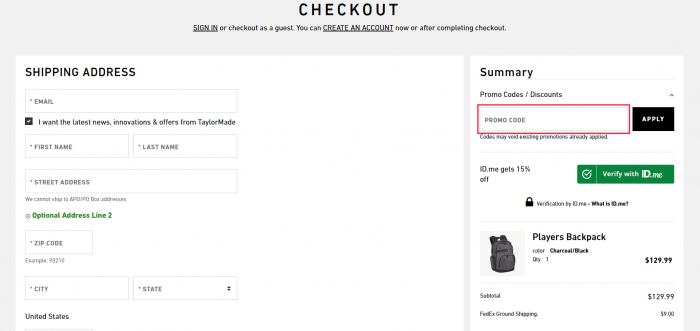A screenshot captures a typical e-commerce checkout page, characterized by its minimalistic, text-based layout. Dominating the top of the page is a pale blue banner with white text that reads "Checkout," accompanied by options for users: "Sign In" or "Checkout as a Guest." The banner also offers the possibility of creating an account either now or after the completion of the checkout process.

On the left side of the page, set against a white background, are standard fields for entering the shipping address—these include text boxes for the email address, name, street address, and other related details.

The right side of the page features a distinct white text box summarizing the order. This summary includes a red-outlined text box labeled "Promo Code" with a black "Apply" button beside it. Another section, highlighting a 15% discount for ID.me members, includes a green "Verify with ID.me" button.

Below this summary is a small photo of a gray "Player's Backpack," priced at $129.99. The item is to be shipped via FedEx Ground, with a note indicating a cost that appears to be five dollars, though the exact amount is slightly unclear due to blurry print. This straightforward page lacks any prominent branding, leaving the identity of the e-commerce company a mystery.